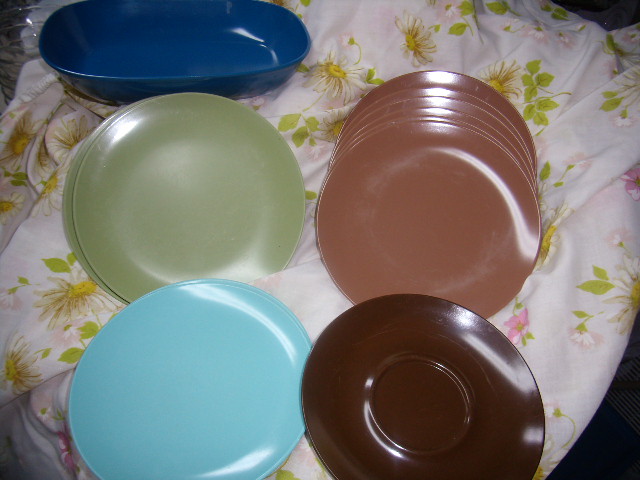In this vibrant color photograph, we're looking downwards from a first-person perspective at an array of crockery arranged on a floral-patterned tablecloth, which features pink and yellow flowers with green leaves. The tablecloth is slightly wrinkled, giving it a casually thrown appearance. 

The crockery consists of various plates and one bowl. In the bottom right corner, there's a dark brown saucer with an inner ring, likely designed to prevent slipping. This saucer, along with the other plates, has a noticeable highlight near the 1-2 o'clock position, reflecting the light source, possibly from a camera flash or overhead light.

To the left of the brown saucer, there's a very turquoise plate. Above this, two lime green plates are stacked, which have a dull, muted army green hue. The largest collection of plates is on the back right, comprising a fanned-out stack of approximately six light brown plates with a reddish tint, described as brick-colored. These segments, coming towards the camera, add a dynamic visual interest. 

In the back left, there's a deep ocean blue oval dish, likely used as a serving bowl with a lip around its edge. Despite their colors being described as dull, the plates appear to be capturing the light well, indicating their smooth surface.

This image showcases a mix of colors and textures, creating a detailed and visually interesting arrangement of everyday items.